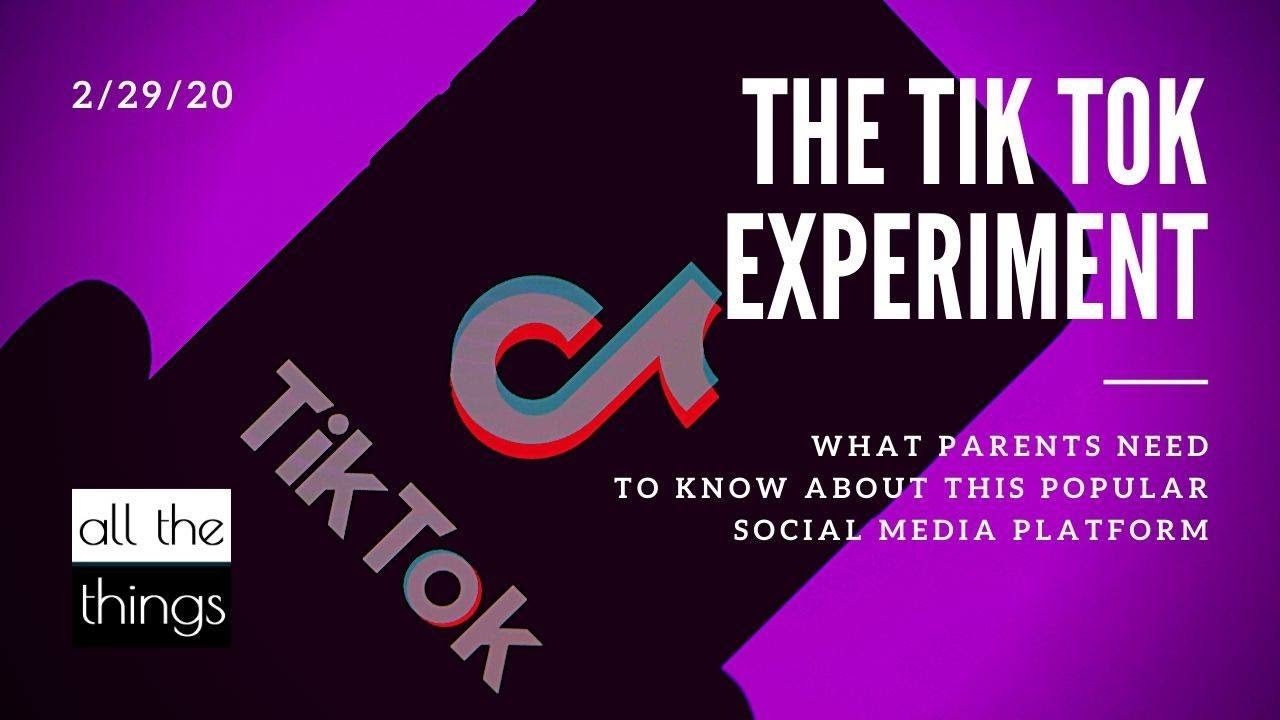This image is a colorful promotional graphic for an event or article related to TikTok, potentially published on February 29, 2020. The top left corner displays the date, suggesting it's an upcoming release or event that aims to generate interest. The central focus of the graphic is the TikTok logo set against a pink background, with the words "The TikTok Experiment" prominently displayed in large white letters. Beneath the main title, there's a subheading in smaller lettering: "What parents need to know about the popular social media platform." In the bottom left corner, the text "All the Things" appears, likely indicating the name of the organizing entity behind this content piece. Overall, the image serves as an informative teaser for a discussion, article, or podcast aimed at educating parents about TikTok.